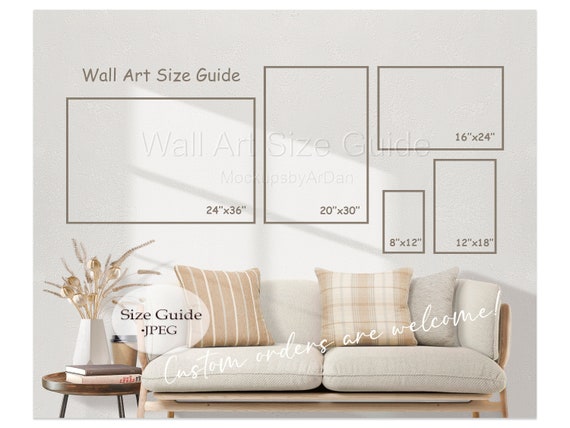This image captures a cozy indoor setting, featuring a couch with white cushions adorned with beige pillows that have white stripes and plaid patterns. The couch, which has a wooden frame, is a mix of white-gray shades and beige, giving it a warm, inviting look. Positioned beside the couch is a wooden side table holding two books, a cup of coffee, and a white vase containing brown and yellowish plants. The background wall is white and prominently displays a wall art size guide with five different size rectangles: 24 by 36 inches, 20 by 30 inches, 16 by 24 inches, 8 by 12 inches, and 12 by 18 inches. The guide is labeled in two different fonts, adding a decorative yet informative touch to the composition.